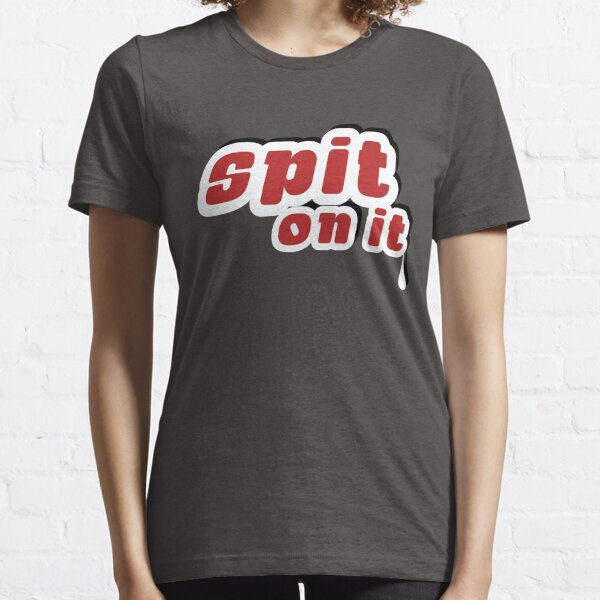This photograph features a female model standing in front of a rustic white brick wall, freshly painted. The model is shown from just above her wrists to her mid-neck, and we can see a bit of her curly hair. She is wearing a short-sleeve, dark slate gray shirt with creative text on it. The text is in a bold red font with a thick white outline and a black shadow, creating a 3D effect. The shirt displays the phrase "spit on it," with "spit" being larger and more prominent than "on it," and a white droplet dripping off the end of the T in "it." The image focuses on the shirt and the details of the text against the plain background.